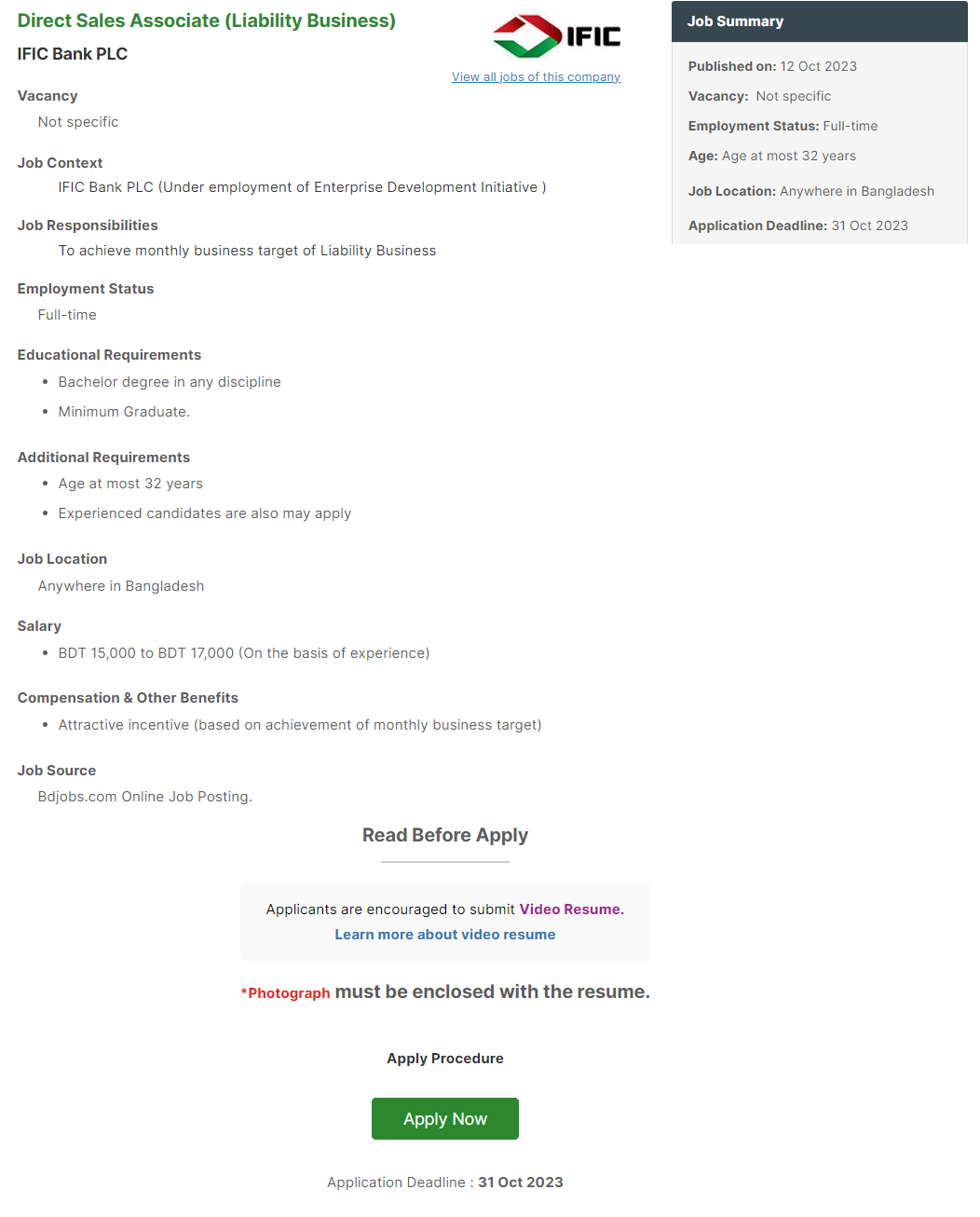The image features a white background with various text elements and sections described in detail. In the upper left corner, there is green text that reads "Direct Sales Association" with "Viability Business" enclosed in parentheses. Adjacent to this, there is a distinctive black logo with the acronym "IFIC," underneath which there is a underline in blue that reads "View All Jobs in this company."

To the right, there is a grayish border containing text segments in various shades of gray. The section titled "Job Summary" includes details in a lighter gray background with black text which states: "Published on 12 October 2023," followed by "Vacancy Notice: Not Specific," "Employment Status: Full Time," "Age: At most 32 years," "Job Location: Anywhere in Bangladesh," and "Application Deadline: 31 October 2023."

Beneath this summary, the green text "IFIC Bank PLC" is noticeable. Further down, additional job details are outlined as follows: "Vacancy: Not Specified," "Job Context: IFIC Bank PLC, Under Employment of Enterprise Development," "Job Responsibilities: Achieve Monthly Business Target of Viable Businesses," "Employment Status: Full Time," "Educational Requirements: Bachelor's Degree in Any Discipline (Minimum Graduate)," "Additional Requirements: Age at most 32 years, Experience Candidates may also apply," and reiterated "Job Location: Anywhere in Bangladesh." The job salary range is indicated as "BDT $15,000 to BDT $17,000 based on experience."

At the bottom of the image, there is a green rectangular button with white text that says "Apply Now," and once more, the application deadline is reaffirmed: "Application Deadline: 31 October 2023."